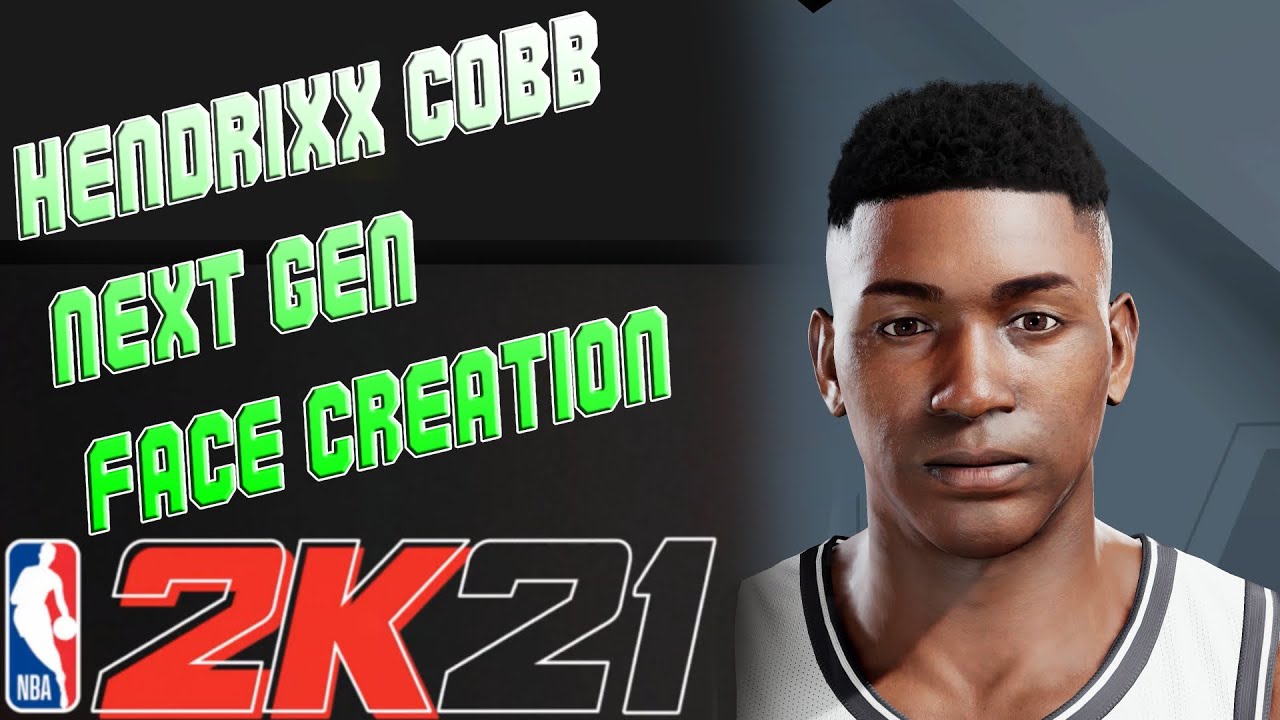This image serves as a YouTube thumbnail for a video focused on creating a custom player in NBA 2K21. The central figure is a young black male in his 20s or 30s, adorned in a striking white jersey with black accents. The player is set against a textured blue-gray background, enriched with overlaying darker patterns. On the left side, a blurred black box appears with text overlay, featuring the title "Kendrick Cobb Next Gen Face Creation" in a dynamic, diagonal font. The text is presented in a captivating gradient of white and neon green, angled towards the top of the image. Below this, iconic logos appear: the red, white, and blue NBA basketball logo, followed by the red and black 2K21 logo, signifying that this content pertains to the NBA 2K21 video game. This thumbnail effectively previews the video content, showcasing the custom player and the title.